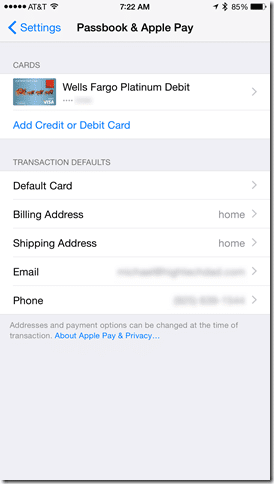The image is a screenshot from a mobile phone, displayed in portrait format, meaning it is taller than it is wide. At the top left corner, there are five black dots adjacent to the 'AT&T' carrier label and a signal strength icon. Centrally placed at the top, the time is shown as 7:22 AM. On the right side of the status bar, there are several icons: an arrow pointing northeast, a Bluetooth symbol, '85%' indicating the battery charge, and a nearly full battery icon reflecting the same charge level.

Beneath the status bar, there is a blue backwards arrow followed by the word 'SETTINGS' also in blue. Centered on the screen, 'Passbook & Apple Pay' is written in bold black text. Below it, a grey strip runs horizontally with the word 'CARDS' displayed on it.

Under the 'CARDS' section, there's an image of a Wells Fargo Platinum Debit card against a blue background. The card details are partially obscured with four asterisks and blanked-out numbers, an arrow pointed to the right is also present. Next, in bold blue lettering, it says 'ADD CREDIT OR DEBIT CARD.'

Further down, another grey banner reads 'TRANSACTION DEFAULTS' in capital thin grey lettering. Below this, there are several line items: 
1. 'DEFAULT CARD' followed by a right arrow.
2. 'BILLING ADDRESS' showing 'HOME' and a right arrow.
3. 'SHIPPING ADDRESS' also displaying 'HOME' and a right arrow.
4. 'EMAIL' and 'PHONE' both with their details blanked out.

At the very bottom of the screen, a grey box contains the text, 'ADDRESSES AND PAYMENT OPTIONS CAN BE CHANGED AT THE TIME OF TRANSACTION.' Beneath this statement, 'ABOUT APPLE PAY AND PRIVACY...' is presented in bold blue text, indicating a clickable hyperlink that likely leads to further information.